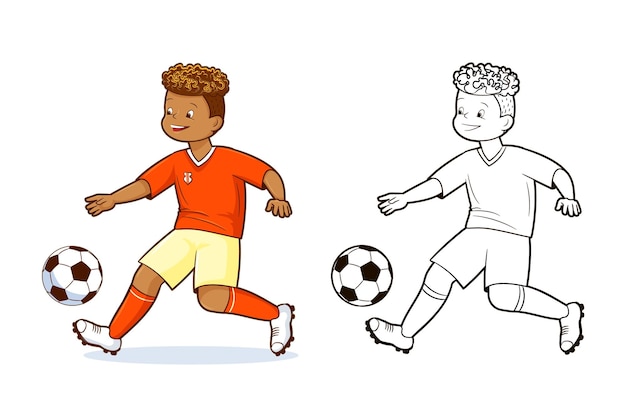The composition features two images of the same boy engaged in playing soccer, both depicted against a white background. On the right is a black-and-white ink sketch, while the left side showcases a fully colored version. The young boy, of Afro-American descent with brown skin and dark brown hair, is captured in motion, in the act of kicking a soccer ball with his right leg and his hands outstretched, displaying a joyful smile. He is dressed in an orange V-neck shirt featuring a small logo on his right chest, yellow shorts, orange knee-high socks, and white soccer cleats with black bases. The contrasting portrayal highlights the lively and detailed color version set against the monochromatic sketch, both illustrating the boy's dynamic action and cheerful expression.